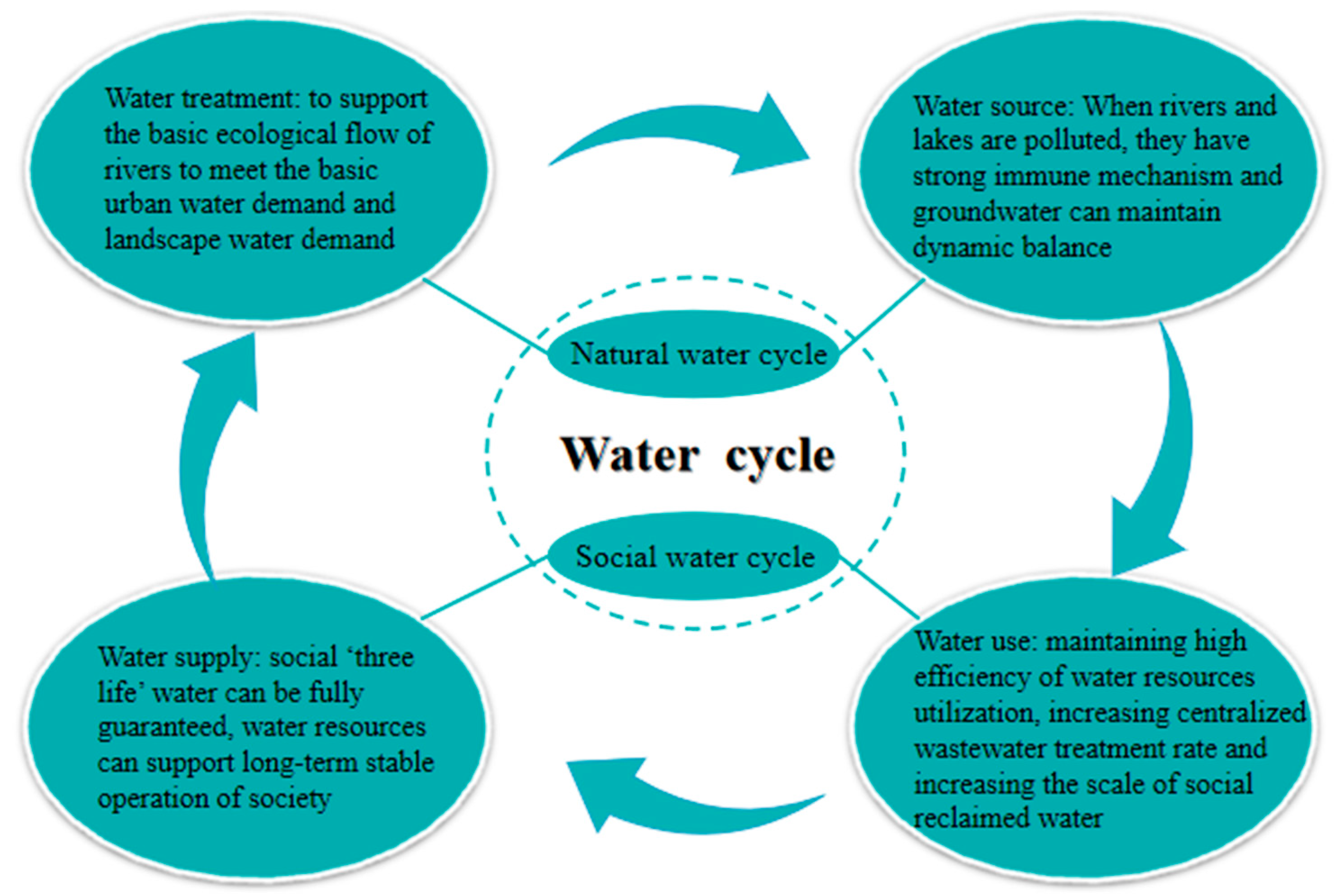This detailed image is a diagram of the water cycle, both natural and social, presented against a white background. Central to the diagram is a black text label "Water Cycle," further divided into sections labeled "Natural Water Cycle" and "Social Water Cycle" within a central circle. Surrounding this central circle are four aqua blue bubbles symmetrically positioned, connected by clockwise arrows, illustrating the process flow of the cycle.

The top-left bubble reads: "Water treatment to support the basic ecological flow of rivers, meeting the basic urban and landscape water demand." The top-right bubble states: "Water source: When rivers and lakes are polluted, they have strong immune mechanisms, and groundwater can maintain balance." The bottom-right bubble explains: "Water use: Maintain high efficiency of water resources utilization, increasing centralized wastewater treatment rate, and scaling up social reclaimed water." Finally, the bottom-left bubble, labeled "Water supply," asserts: "Social lifewater can be fully guaranteed, ensuring water resources can support long-term stable societal operations."

The diagram uses a color palette of blue, green, white, and black, with aqua blue arrows and text on an aqua background for the bubbles, emphasizing clarity and connectivity in the cyclical process. The balanced placement of the bubbles and the consistent use of colors contribute to an organized representation of the complex yet essential system of water circulation and management.